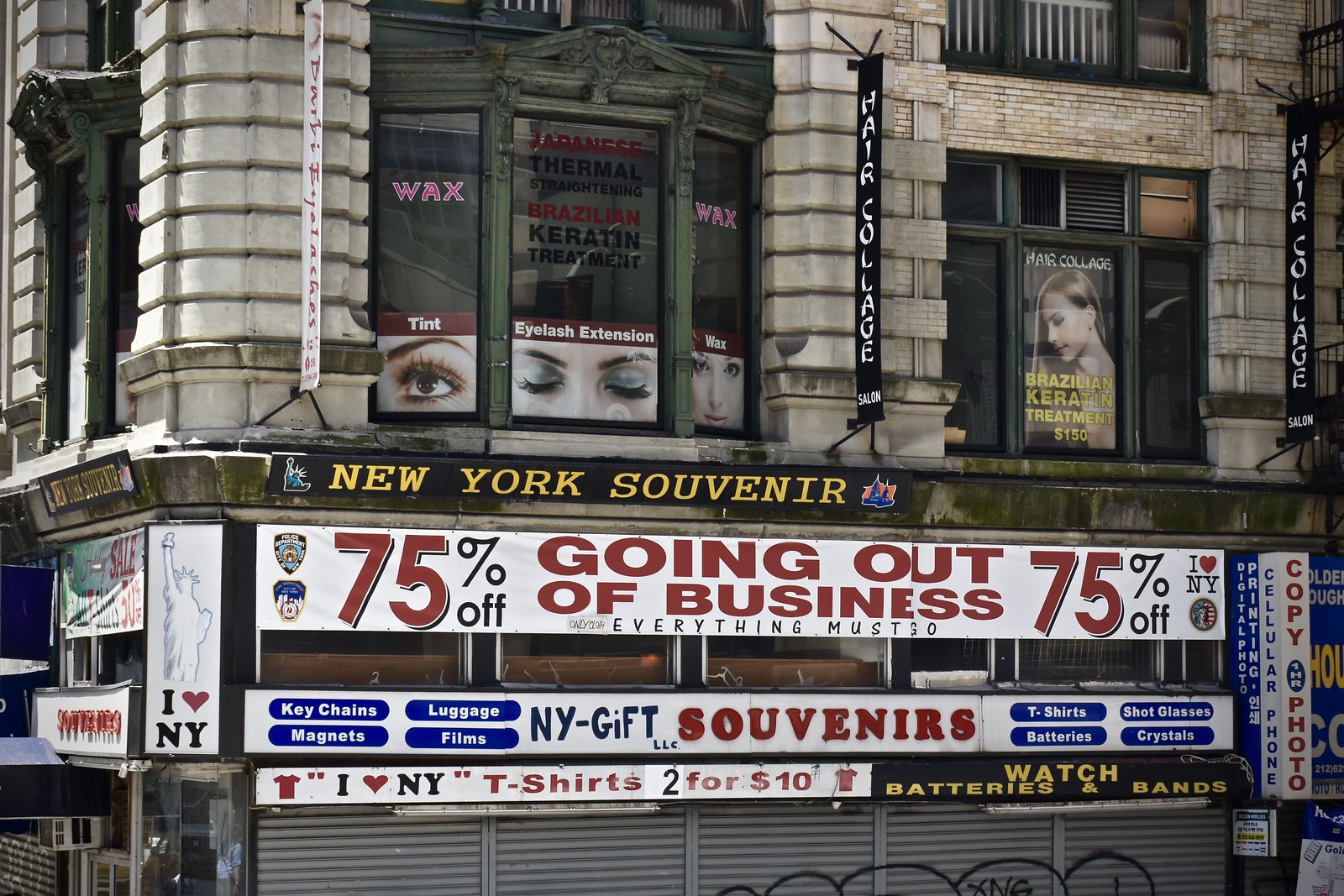This photograph captures a quintessential New York city street scene dominated by an older, gray limestone building with green-trimmed windows. At the building's base is a prominent New York souvenir shop, displaying a large white banner with blue and red accents declaring, "75% off, going out of business, everything must go." Below this, another sign prominently advertises "New York Gifts Souvenirs," alongside offerings such as keychains, magnets, luggage, film, and I Love New York t-shirts, two for $10. The storefront, shielded by closed, graffiti-marked metal sliding doors, also mentions watch batteries and bands. Above the souvenir shop, the second floor showcases large glass windows adorned with images of women's eyes and faces, advertising services like Japanese Thermal Straightening and Brazilian Keratin Treatment under the name "Hair Collage." This detailed street-level view encapsulates the bustling, multifaceted nature of New York City's commercial districts.